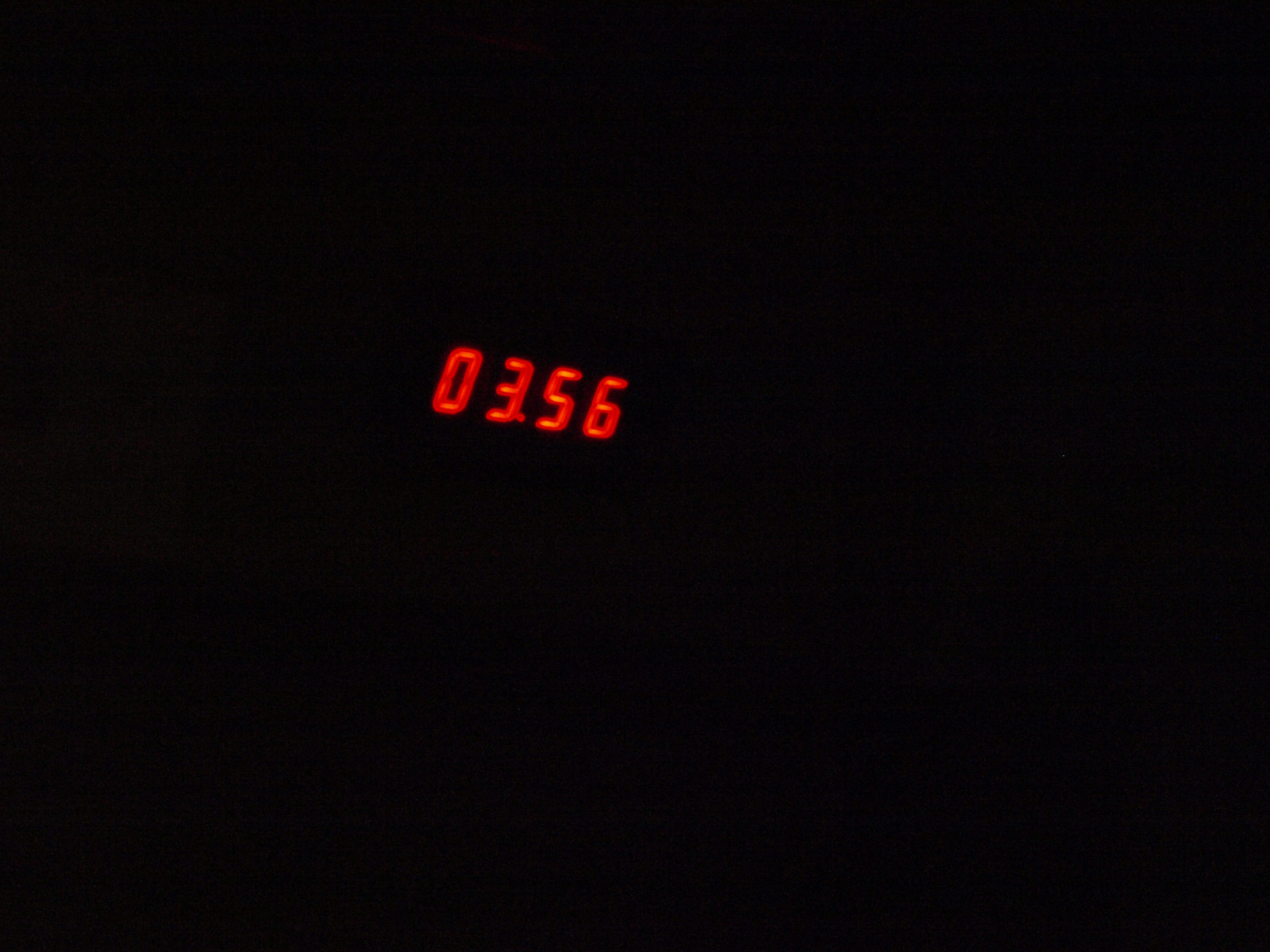The photograph features a predominantly black background, devoid of any discernible elements other than a series of red digits prominently displayed near the center. These digits, "03.56," are reminiscent of those found on an alarm clock, glowing with a faint blur yet remaining legible. Positioned slightly to the left, the numbers are tilted downward at an angle, adding a sense of dynamic tension to the otherwise stark and minimalistic composition. The darkness envelops the image, focusing the viewer's attention solely on the glowing numerals amidst the void.